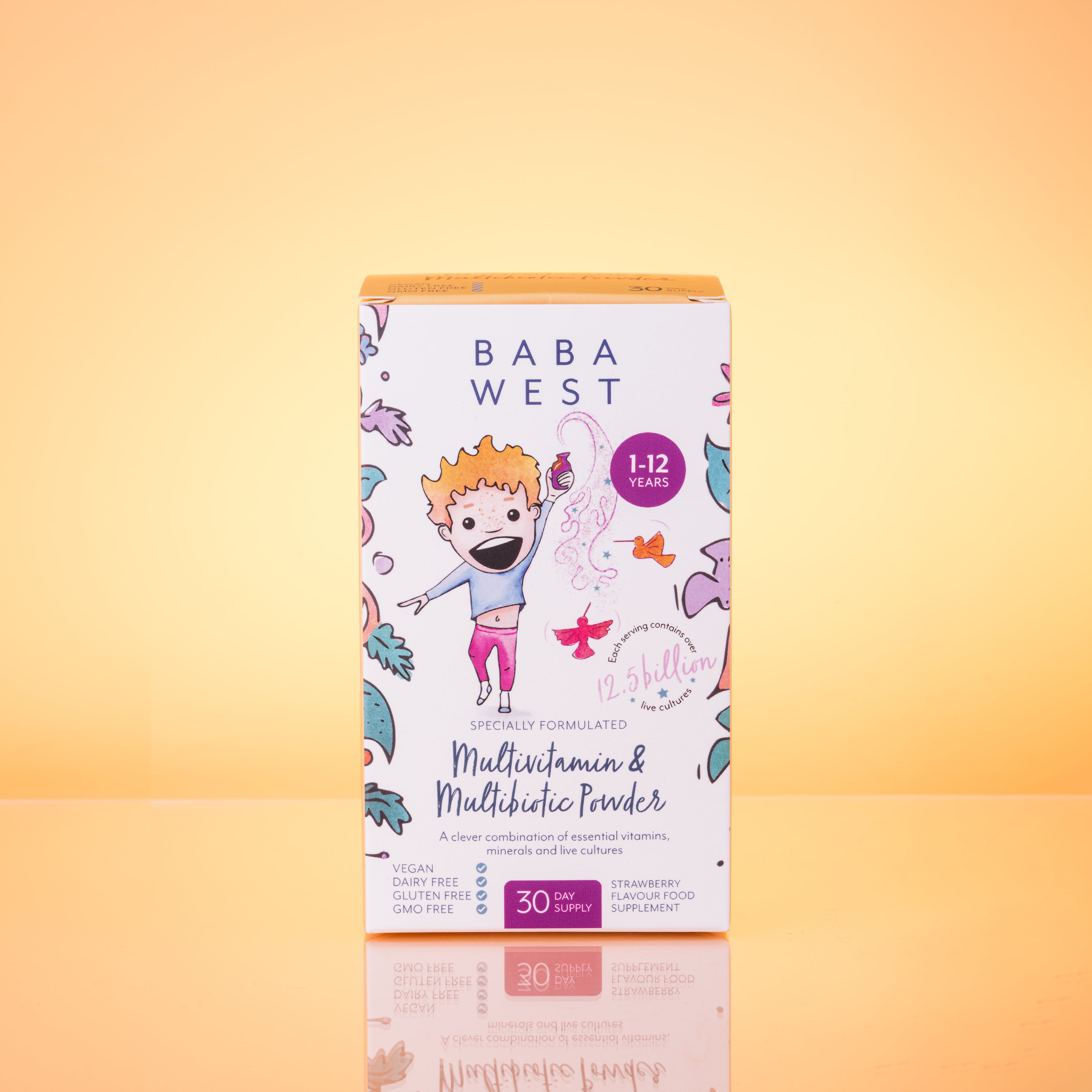The image displays a professionally staged photograph of a multivitamin and multibiotic powder product package from Baba West. The background is a light peach-orange hue, providing a contrasting backdrop to the predominantly white rectangular box with an orange top. Prominently featured on the box is a cartoon of a small child with blue hair, a blue shirt exposing his belly, and pink pants, holding a bottle above his head from which colorful powder or smoke in hues of purple, blue, red, pink, and peach erupts. Overlaying this image, in blue text, the brand name "Baba West" is displayed, alongside a purple circle stating "1 to 12 years." Additional details include orange and pink birds around the emerging powder and text indicating that the product contains 12.5 billion cultures. The box further advertises that it is a specially formulated multivitamin and multibiotic powder, highlighting its vegan, dairy-free, gluten-free, and GMO-free properties. Touted as a 30-day supply of strawberry-flavored food supplement meant to support children's gut health and overall wellness, this clever combination of essential vitamins, minerals, and live cultures is clearly aimed at parents seeking a functional health product for their children aged one to twelve years.